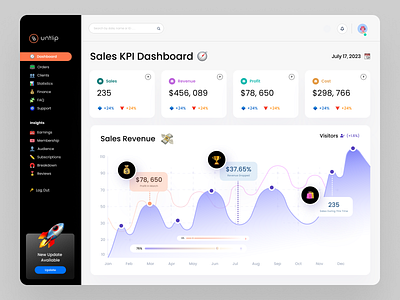The image is a detailed screenshot of a Sales KPI Dashboard, a software program used at work. The dashboard has a white background with black letters at the top stating "Sales KPI Dashboard." It features four equal-sized boxes displaying numeric values: $235, $456,089, $78,650, and $298,768. Below these boxes is a larger rectangular box titled "Sales Revenue," accompanied by a money icon. This section contains a graph depicting the fluctuating trends of sales, with a hill-like structure shown in purple and marked with purple dots at the peaks. On the left side, there is a vertical black menu highlighted in orange at the top, which includes a dropdown list of options and a rocket ship icon at the bottom. A blue clickable section for more information is also present. The four numbered boxes have headings in various colors—green, purple, light green, and orange—describing the data they represent. The Sales Revenue graph displays dates on the left and bottom axes, charting the sales trends from left to right.